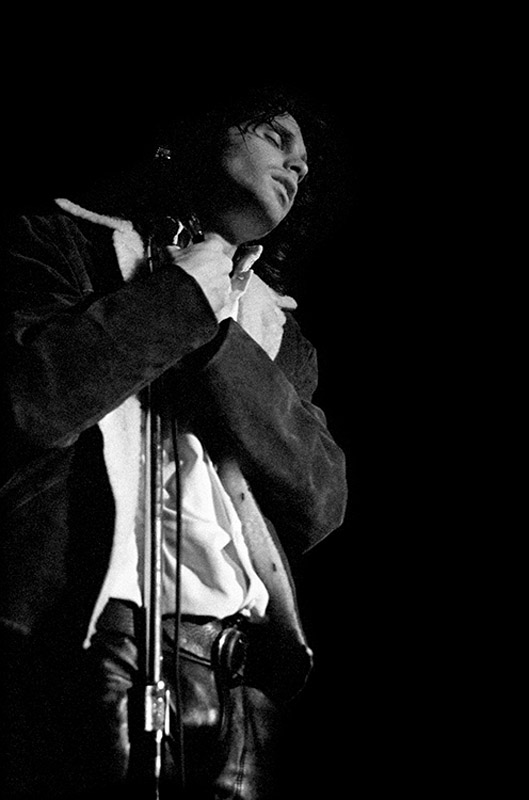In this striking black-and-white photorealistic image, a singer stands on what appears to be a stage, passionately clutching a microphone stand. His head tilts to the side and his eyes are closed, immersed in an overwhelming emotion. The gentleman boasts medium to long, wet, curly hair that falls over his face and possibly an earring glinting on the right side. He dons a dramatic outfit consisting of black leather pants, a fancy large belt buckle, and a black jacket lined with soft, white fur, over a white collared button-up shirt. The background is pitch black, emphasizing his presence and adding to the intensity of the moment captured.